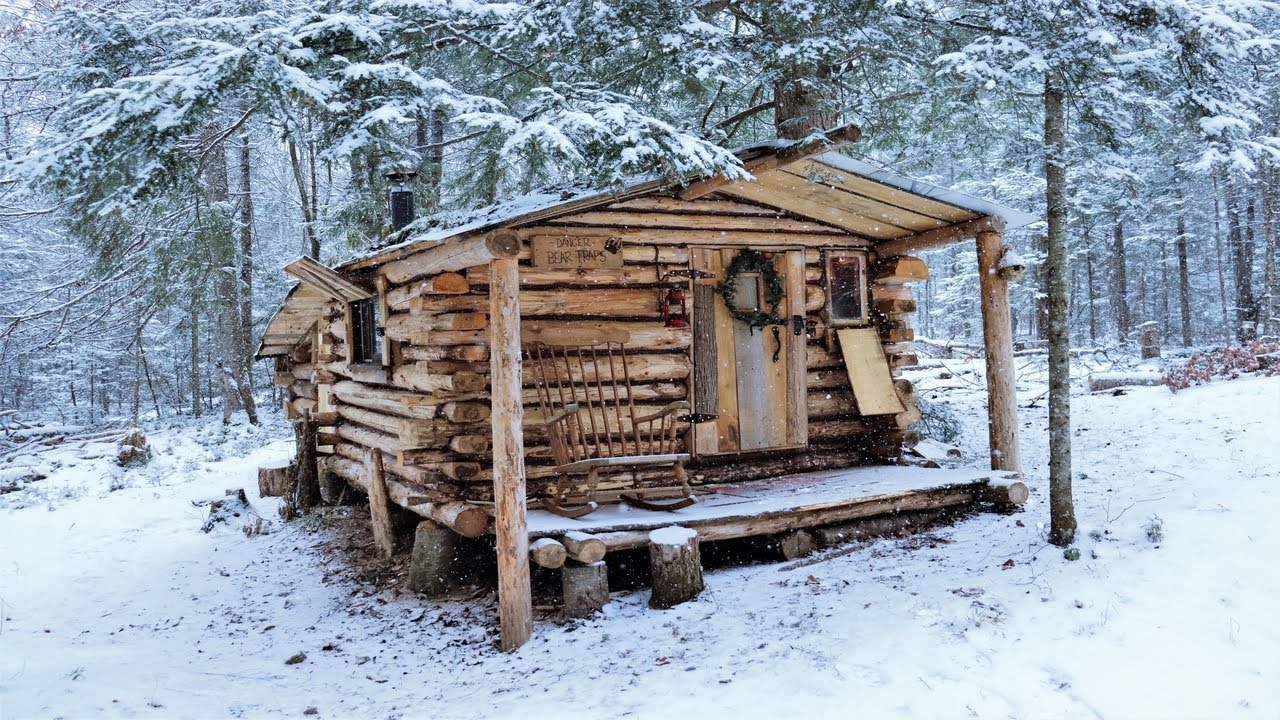The photograph showcases a small, rustic log cabin situated in a snowy field amidst a forest. The cabin is constructed from light-colored logs that appear weathered and varied in length, contributing to its charmingly rough-hewn appearance. A wooden rocking chair sits on the front patio, which itself looks slightly uneven as it's supported by logs of differing sizes. At the center of the cabin's front, a plain rectangular door adorned with a wreath stands out. A wooden sign bearing a "Danger Bear Traps" warning, along with a bear paw print, is prominent on the top left part of the cabin. The cabin, likely one story with one or two rooms, features small windows on either side of the door. The ground surrounding the cabin is completely covered in snow. In the background, the forest trees are blanketed with snow, adding to the wintery ambiance of this secluded woodland retreat.